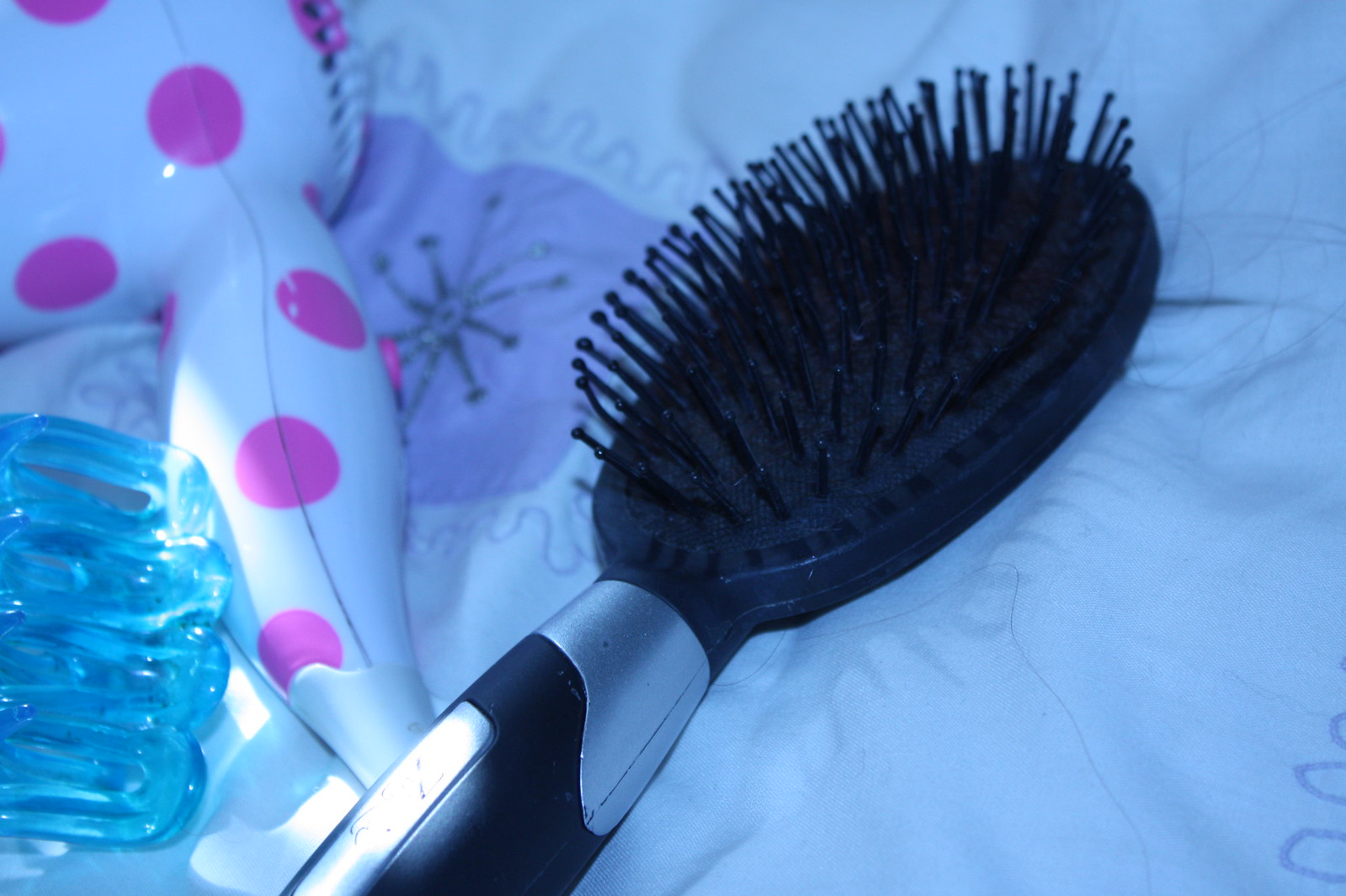This close-up photograph features hair tools neatly arranged on a slightly wrinkled, white bedspread adorned with a colorful pattern of starbursts, squiggles, and squares in lavender, blue, pink, and black. The prominent object in the center is a black hairbrush, characterized by an oval-shaped pad filled with black bristles topped with small protective balls. This brush also includes a distinctive metallic silver section running down its handle. To the left of the hairbrush, we find a white electronic hairdryer with whimsical pink polka dots, its handle and a portion of its head visible in the frame. Additionally, there is a slightly blue, translucent hair clip positioned near the hairdryer. The appearance of light brown hair tangled within the hairbrush's bristles adds a touch of realism to this everyday scene.